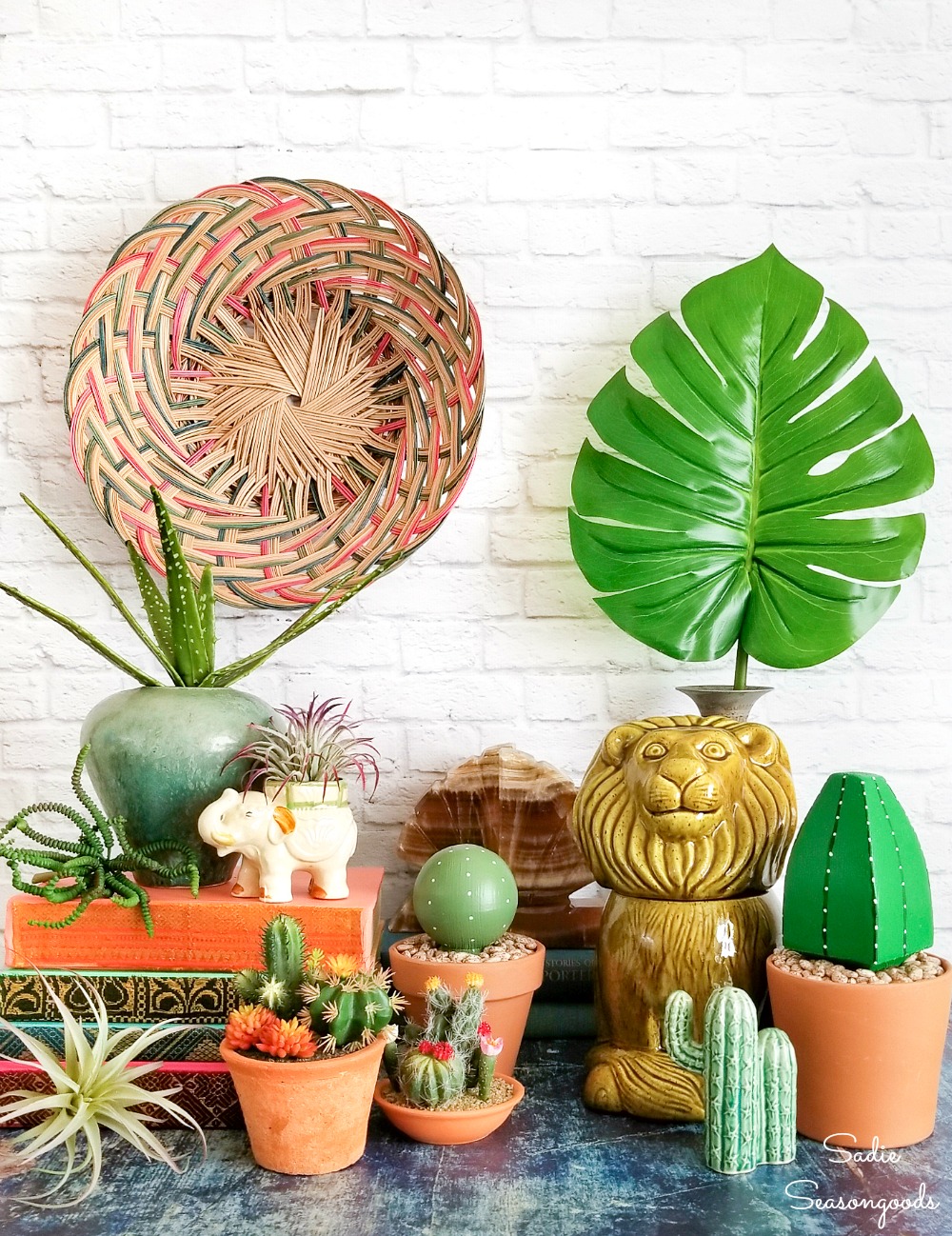The staged photograph showcases a vibrant and eclectic indoor garden display set against a white painted brick wall. Central to the scene are two potted plants on a table, one short and bushy and the other tall with larger leaves, both exuding lush green hues that provide a refreshing contrast to the predominantly brown and earthy tones. Hanging behind the plants is a colorful wicker basket in green and blue, adding a splash of vibrancy to the display.

Among the decorative items, a white ceramic elephant planter with flowers stands out, along with an ornate, golden, ceramic lion figurine that adds a touch of grandeur. A large, artificial leaf emerges from a tall vase situated behind the lion, contributing to the botanical theme. The display also features various other elements like woven plants and cacti, hinting at a potential garden-like product advertisement, possibly for a brand called Sadie's Seasoned Goods, as indicated by a sign in the lower right corner of the image.

The scene is set on blue-stained wooden flooring, which complements the overall color palette. Additional details include a smaller woven basket and what appears to be statues or fake plants of cacti, enhancing the garden motif. The display exudes an artistic and curated feel, likely representing a domestic setting such as a living room or a promotional setup for gardening products.